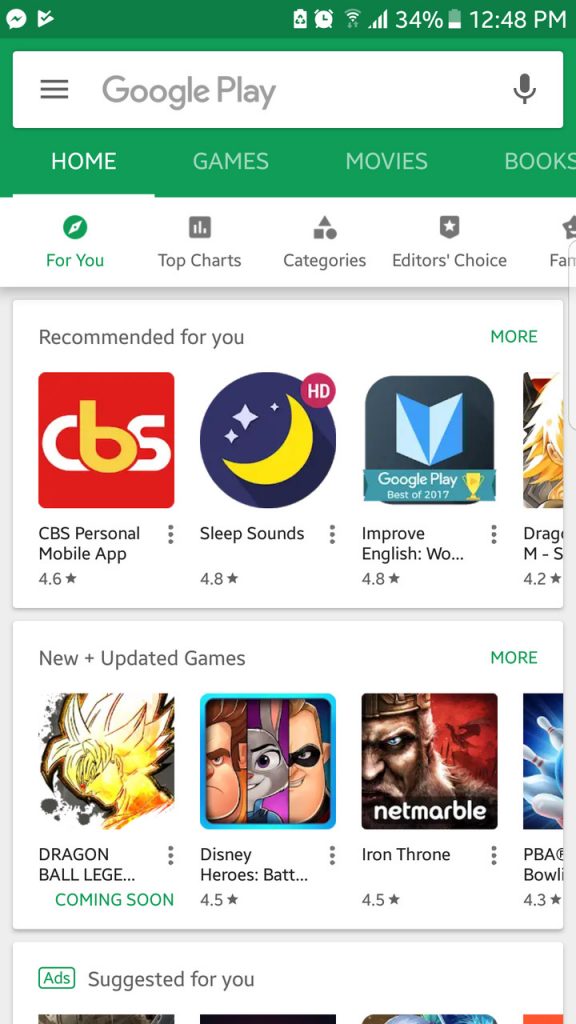A screenshot of a cell phone displaying the Google Play Store interface. At the top, the screen has a green background with white text, including a speech bubble icon with a line through it, indicative of a notification. Other icons displayed include battery saver, alarm clock, Wi-Fi, and cell signal strength, with a battery percentage of 34%.

Below this, a lighter green background features a white search bar for Google Play with a microphone icon on the right. The navigation tabs underneath consist of “Home” in white, and “Movies,” “Music,” “Books” in grey. Beneath these tabs, on a white background, there's a green highlighted “For You” section followed by grey tabs labeled “Top Charts,” “Categories,” and “Editor’s Choice.”

Following this, the screen presents recommended apps which include “CBS Personal,” “Mobile App,” “Sleep Sounds,” “Improve English,” and a partially visible fifth app. Further down, under “New and Updated Games,” featured apps include "Dragon Ball Legends," "Disney’s Hero Battle," and "Iron Throne."

At the bottom of the screenshot, there is an advert marked as “Suggested for you.” The rest of the page is not visible and cut off, awaiting further interaction. The countdown at the end marks the end of this description, followed by a light-hearted "3, 2, 1, Blast Off!" indicating the transition to the next task.